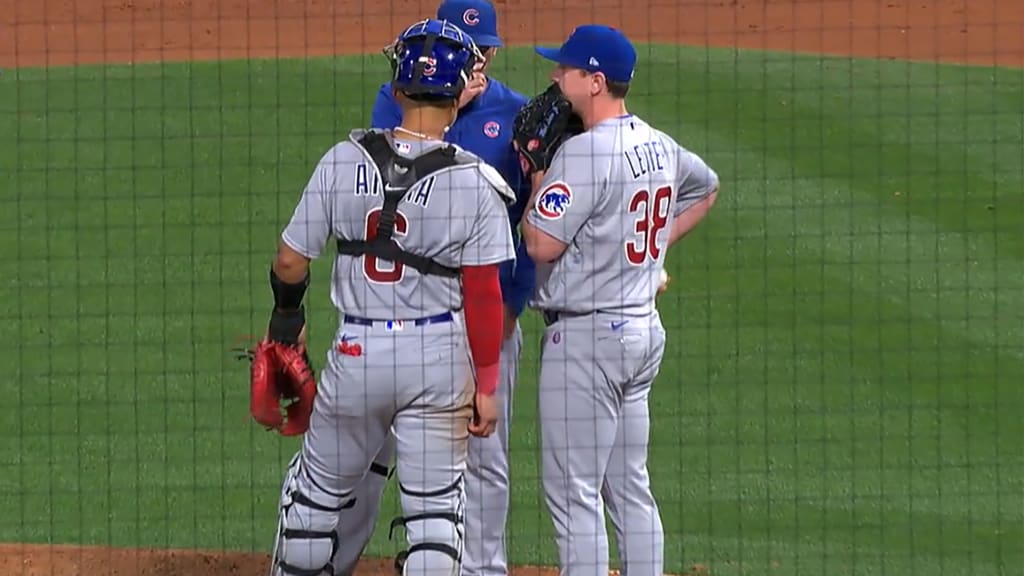The image is a horizontally aligned rectangular photograph taken through a net that creates a grid pattern across the entire scene. It captures three men closely conversing on a baseball field. Two of the men are baseball players wearing gray uniforms with their backs to the camera. The player on the left, identified as the catcher, is wearing knee guards, a red glove, and a helmet, with the number 6 in red on his uniform. The player on the right, number 38, is the pitcher and is wearing a blue Cubs cap adorned with the Cubs logo. Both players' uniforms display red numbers. The third man, positioned between them and slightly facing toward the camera, is the coach. He is dressed in a blue polo shirt and a matching Cubs cap marked with a "C". They are standing on the pitcher's mound, surrounded by the green turf of the field and some visible brown dirt beyond it, likely indicating the area around second base. The imagery suggests a moment of strategic conversation, possibly addressing the pitcher's performance during the game.